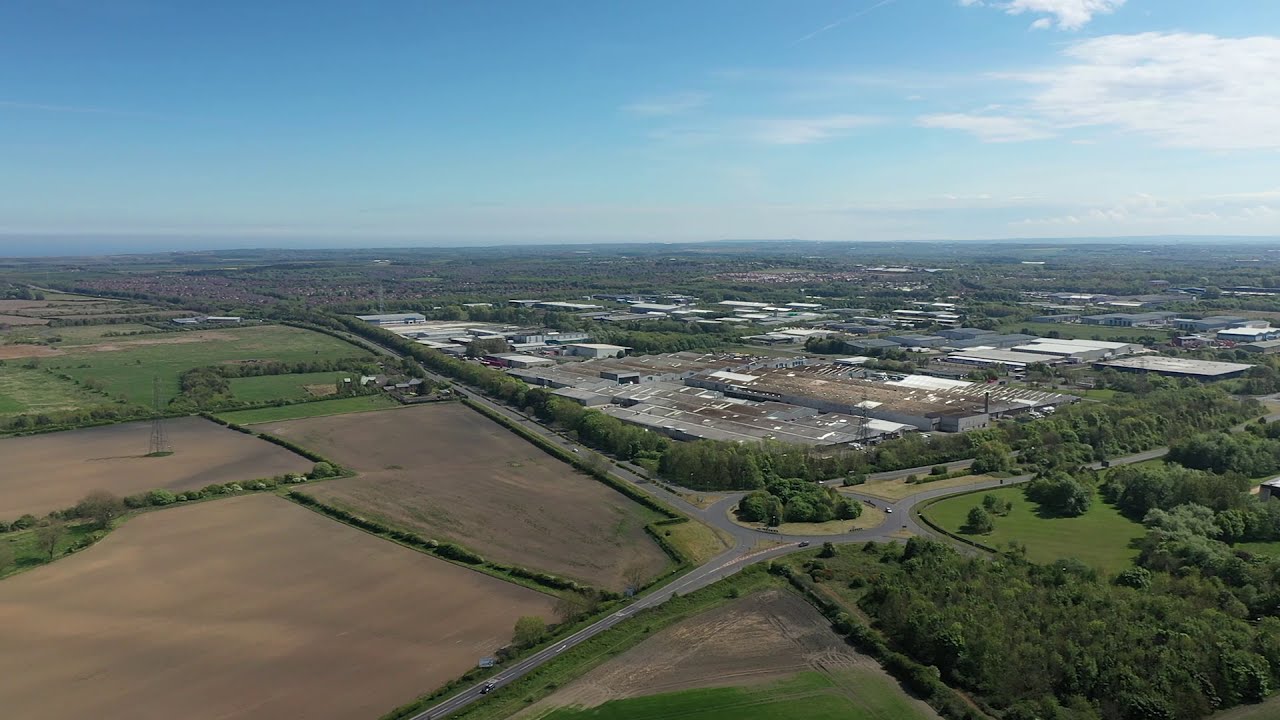This highly detailed aerial photograph, taken from drone height, showcases an expansive terrain with varied features. In the foreground, the left side of the image displays two large, barren fields of red dirt, possibly designated for future agricultural use or construction. Adjacent to these dirt patches is a green pasture that extends towards the horizon. Dominating the central part of the photograph is a significant man-made structure comprising a large gray area with scattered white buildings, hinting at an industrial or agricultural complex. Cutting diagonally through this scene at a 50-degree angle is a gray paved road leading to a prominent circular intersection, or roundabout, which features an island of green trees at its center. To the bottom right, the landscape transitions into dense green forested areas with trees and bushes. Above the complex, the photograph captures a sprawling view of fields and forested regions extending into the distance under a light blue sky adorned with wispy white clouds on the upper right. The scene melds rural and industrial elements, encapsulating a blend of natural and human-altered landscapes.